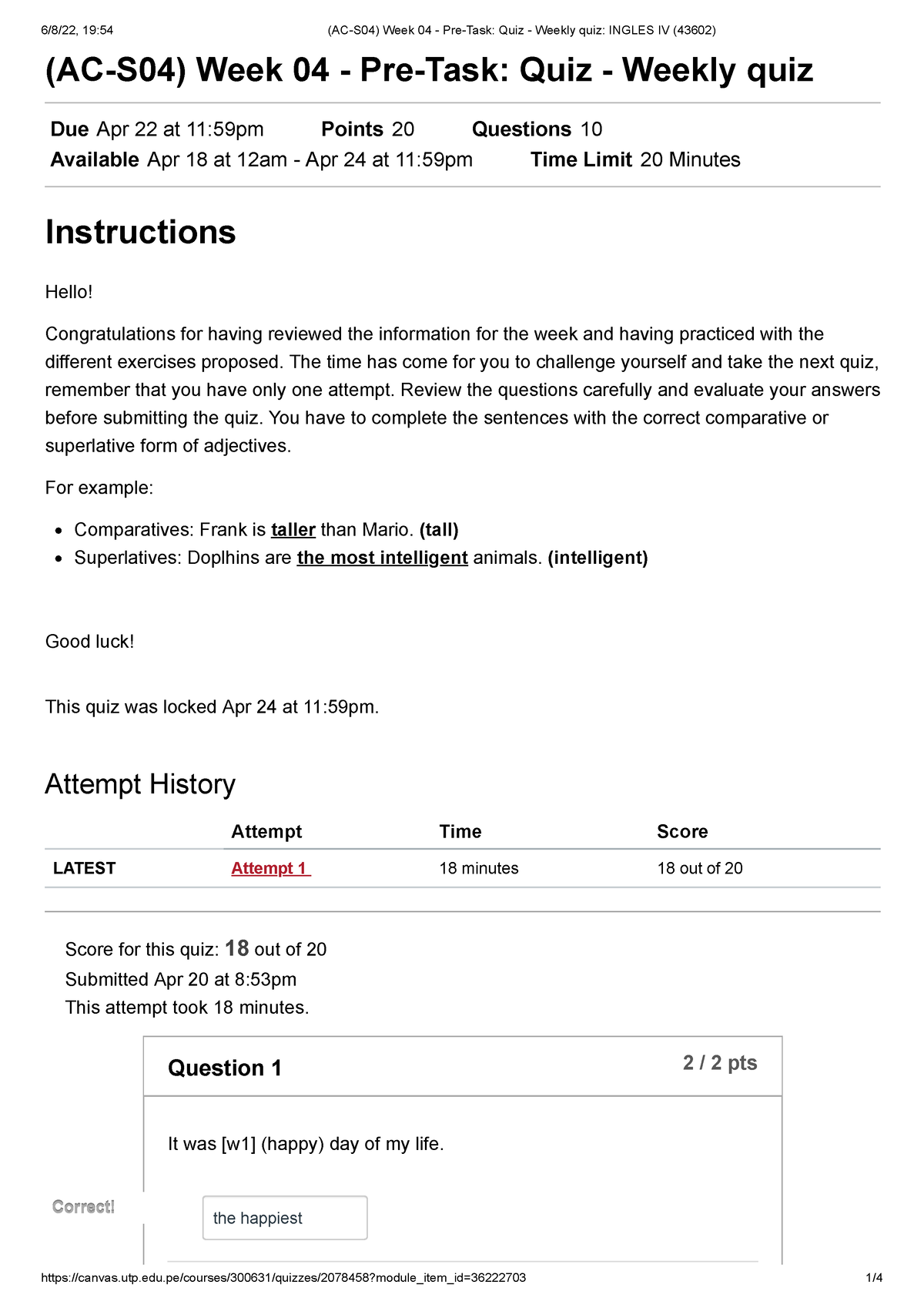**Caption:**

This image displays an online quiz form titled "Week 04 Pre-Task - Weekly Quiz" for an AC SO4 course. The quiz is due on April 22 at 11:59 PM, offering 20 points across 10 questions. It is available from April 18 at 12:00 AM to April 24 at 11:59 PM, with a 20-minute time limit for completion. 

The instructions encourage students to review the week's materials and practice exercises before attempting the quiz. The quiz assesses the correct use of comparative and superlative adjectives. An example for comparatives is "Frank is taller than Manu," where "tall" is highlighted in brackets. An example for superlatives is "Dolphins are the most intelligent animals," with "intelligent" in brackets.

The notice further advises that the quiz permits a single attempt, urging students to review their answers thoroughly before submission. 

The document also provides an attempt history, showing that the latest attempt was completed in 18 minutes, scored 18 out of 20, and was submitted on April 20 at 8:53 PM. The quiz was accessible until April 24 at 11:59 PM.

Additionally, the image includes the first question of the quiz, which shows a sentence with a blank followed by the phrase, "WF happy day for my life," implying the expected correct answer is "the happiest day."